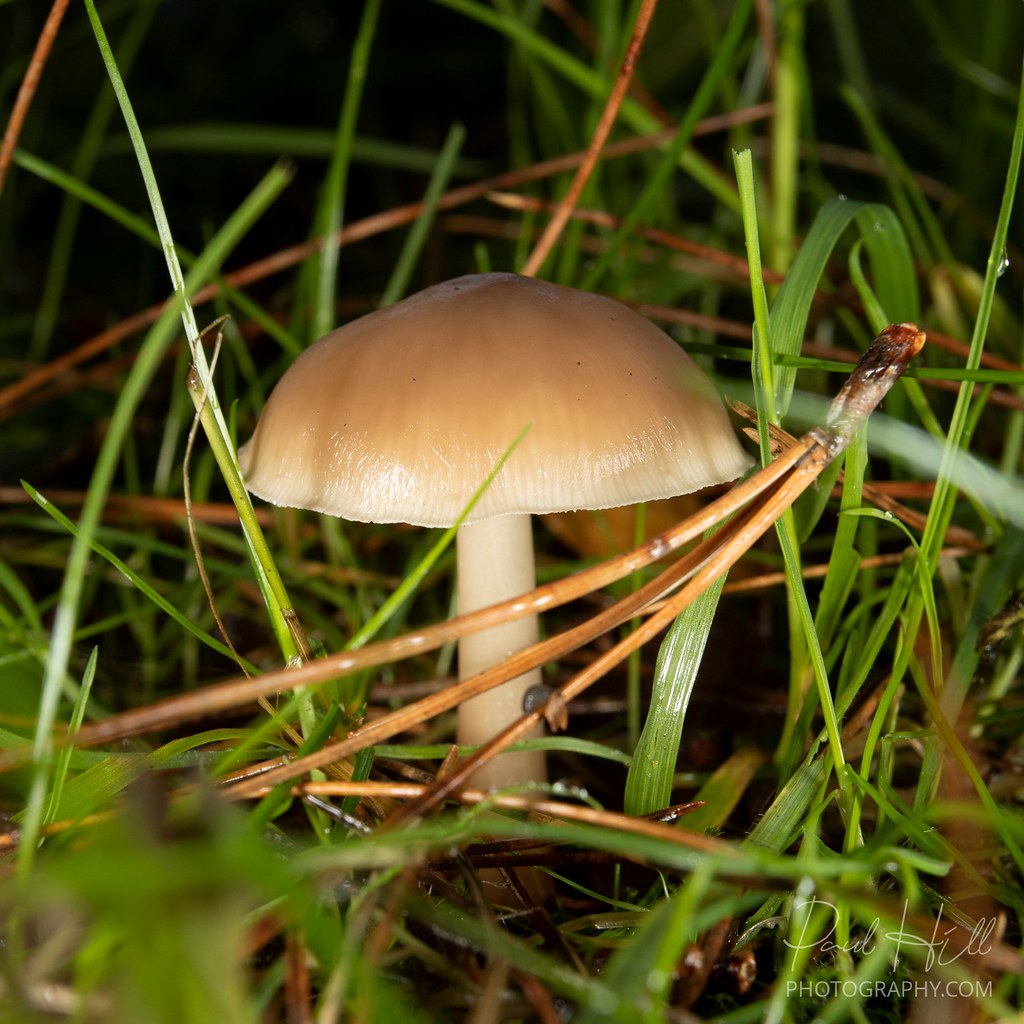In this color photograph, taken by Paul Hill Photography.com, a single mushroom stands prominently in the middle of a garden or grassy field. The mushroom features a slender white stem supporting a bowl-shaped cap that transitions from a reddish-brown at the top to a lighter hue toward the bottom. The scene is depicted with lush green grass blades and interspersed brown twigs and leaf stems crisscrossing in various directions. A small bug can be seen perched on one of the grass blades to the left of the mushroom. The background presents a dark reddish tone, enhancing the contrast and focus on the damp-looking mushroom, which appears to be illuminated by a soft light. The photographer has captured the natural details and textures vividly, magnifying the elements close to the ground.